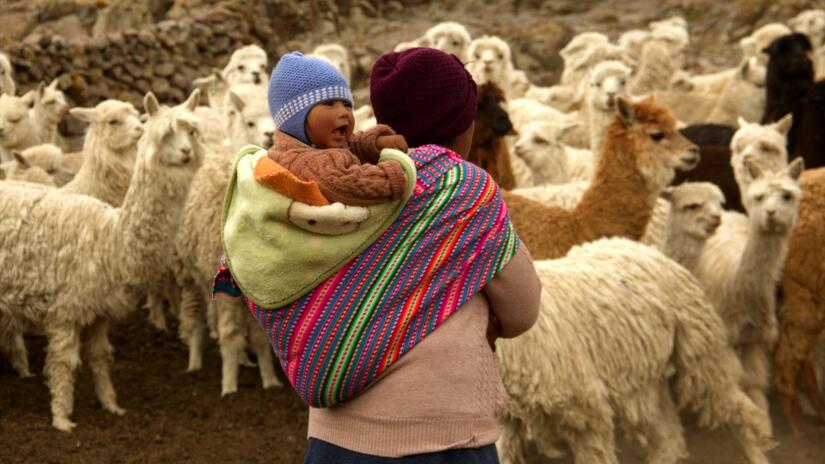In this evocative photograph, a woman, presumably an Andes llama farmer, stands with her back to the camera, tending to her herd of alpacas. The woman is dressed warmly in a pink sweater and a dark purple beanie hat, suggesting a chilly climate. Draped around her shoulders is a brightly patterned sling with stripes of red, blue, green, and purple. Inside the sling, a baby, about three years old, nestles comfortably, swathed in a green blanket and wearing a brown sweater along with a light blue beanie hat.

The herd of alpacas, predominantly white and shaggy, crowds around her in a dense cluster. Among them, a few stand out with their different fur colors—two or three are brown, and one is black. Intriguingly, while most of the alpacas gaze intently at the woman, one near her seems to avert its eyes, looking off to the side as if avoiding eye contact. In the background, a lichen-covered stone wall, likely made from clearing the field, stretches across what appears to be an uphill slope, further anchoring this scene in a pastoral, rugged landscape that hints at South America, possibly Peru. The overall scene is rich with textures, patterns, and a sense of life closely tied to the land.